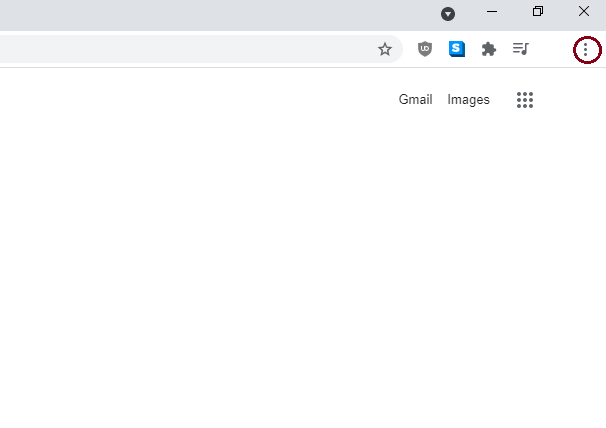This image is a partial screenshot with a white background. The visible portion shows the upper right-hand corner and the top section of a browser window. The top border of the browser is a very light gray color, and in the upper right-hand corner, there is a small "X" icon, which is typically used to close the tab.

Beneath the "X" icon, there are a few other icons. One is a blue square with the letter "S," indicating Skype. Another icon, which appears to be for a music site, features three gray horizontal lines and a musical note.

In the main part of the screenshot, the background remains completely white, except for a small section in the upper right-hand corner. Here, the word "Gmail" is displayed in gray font, next to the word "Images." Additionally, there is an icon consisting of nine small squares grouped together, resembling a grid.